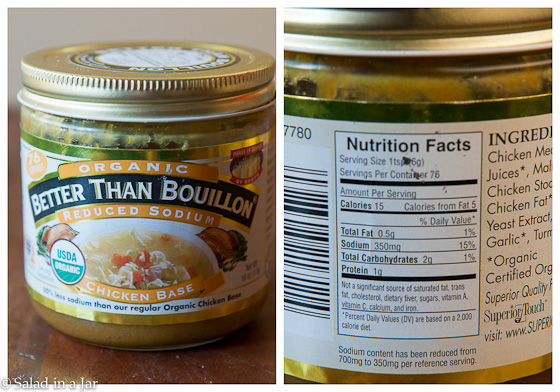The image is a split-screen showcasing both the front and back of a product labeled "Organic Reduced Sodium Better Than Bouillon Chicken Base". The left side of the image displays the product’s front, highlighting its branding, USDA organic certification, and a lid. A picture of a bowl of soup is prominently featured, emphasizing its culinary application. The right side of the image is a close-up of the nutritional facts, detailing key information such as a serving size of 1 tablespoon, with approximately 76 servings per container. Nutritional details are specified: 15 calories per serving, including 5 calories from fat, 0.5 grams of total fat, 350 milligrams of sodium, 2 grams of total carbohydrates, and 1 gram of protein. Part of the ingredient list is also visible, featuring components like chicken juices and chicken stock.